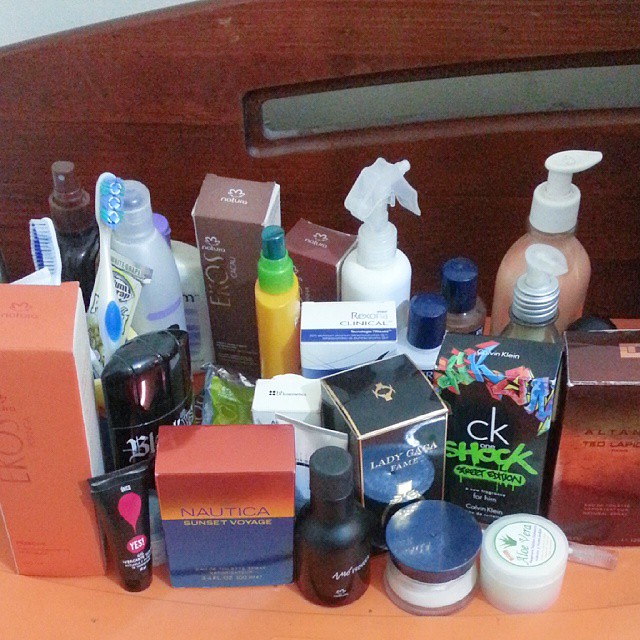A close-up image showcases an assortment of personal care and miscellaneous items meticulously arranged on a vibrant orange surface. Starting from the left, there's an orange box, followed by a small brown tube. Next is a square box that is orange on top and blue on the bottom, labeled "Nautica Sunset Voyage." Adjacent to this is a small brown bottle, a little pot with a blue lid, and a white pot with a white label on top. 

Positioned behind and to the right, there is a brown rectangular box beside a black box adorned with bright green and white lettering that reads "CK Shock." To its right, a reflective black box bears the inscription "Lady Gaga Fame." Two partially obscured white bottles flank a black deodorant-type container. Behind these items stand two white toothbrushes with blue accents. A clear bottle featuring purple details is also visible, with a black bottle with a brown lid situated in the far back left. 

Continuing to the right, a white bottle with a purple lid sits next to a narrow brown box and a bright yellow spray bottle topped with a green cap. In the back, another brown box is seen alongside a white spray bottle. In front, a white box labeled "Clinical" stands out. The display also includes two bottles with blue lids and two hand pumps on the far right. The background reveals part of a wooden frame with a cutout in the middle, set against a white wall.